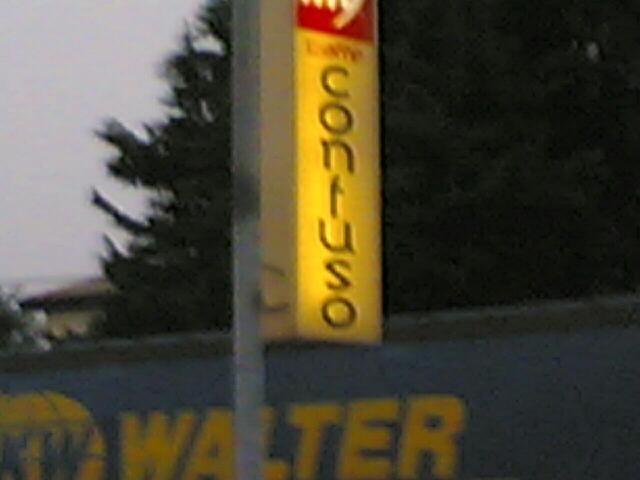This photograph appears to have been taken outdoors on a possibly overcast day, given the dark gray, gloomy sky. Central to the image is a gray pole mounted with a vertical, illuminated yellow sign. At the top of the sign is a red square taking up about a quarter of the sign's space. The text "CONTUSO" is displayed in black vertical letters down the yellow portion of the sign. 

In the background, a billboard with a dark blue background and large yellow letters spelling "Walter" is visible. Next to the word "Walter," there appears to be a logo resembling a yellow globe, complete with latitude and longitude lines. Off in the distance, there are several dark evergreen trees, almost black in appearance, and the roof of a building, possibly a house, with a brown hue is peeking out from beneath the cloudy sky. The overall atmosphere conveys a somber and early evening mood.